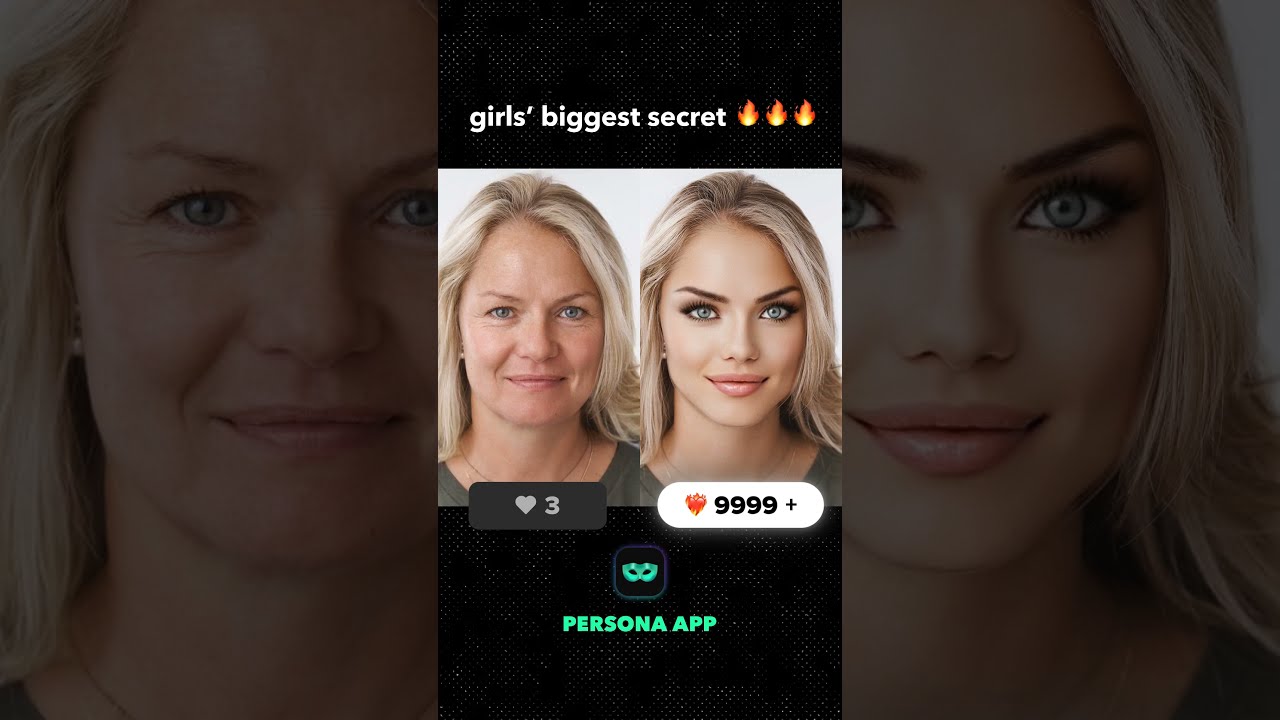The image features a striking before-and-after comparison of a blonde woman to emphasize the transformative power of makeup, potentially enhanced by the Persona app. The top of the image displays the text "Girl's Biggest Secret" in white font, flanked by three fire emojis, against a black background. On the left side of the image, the woman appears naturally, without makeup, with a small heart icon and the number "3" below her face. On the right, she is heavily made up, airbrushed, and almost unrecognizable, with "999+" likes beneath her enhanced visage. The bottom of the image includes the green text "Persona app" alongside a mask icon, suggesting the use of an app to achieve the dramatic makeover. The image features vibrant colors, including black, army green, gray, yellow, orange, red, blue, pink, and white, making it a visually striking depiction of makeup's impact on online appearances.